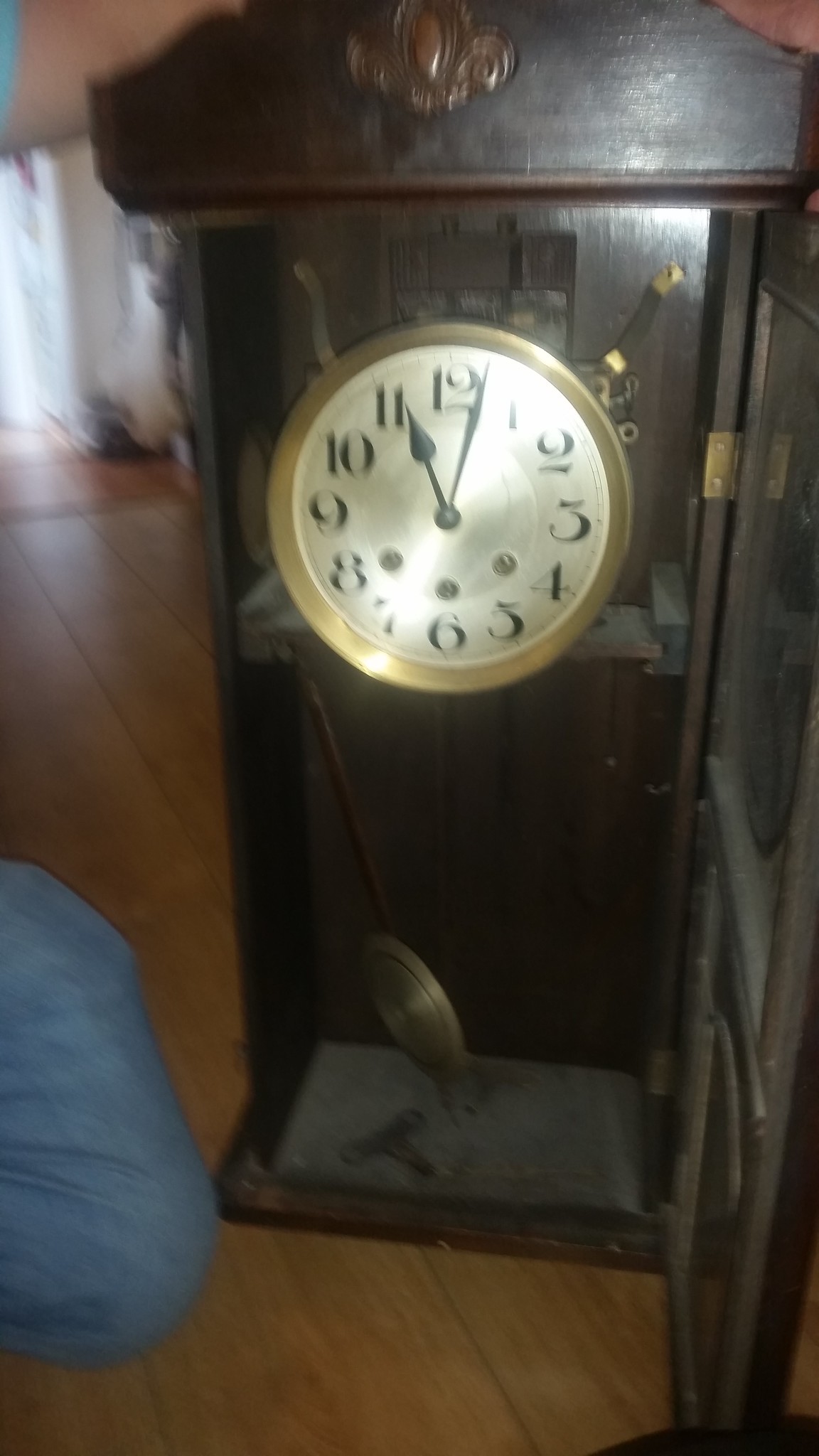This photograph captures a charming, smaller-sized grandfather clock crafted from dark, rich brown wood. The clock's door is open, revealing a golden pendulum swinging below. Enhancing its vintage elegance, the clock face is framed by a golden circle and features a silvery backdrop with bold black numerals. Notably, a layer of dust gathers near the bottom of the clock, indicating its age and use. The clock stands on a mid-toned wooden floor with a slight orangey hue. In the background, to the side of the image, a person's denim-clad knee appears, adding a casual human element to the scene. Gentle blurring in the background suggests a soft light source contributing to the ambient atmosphere.